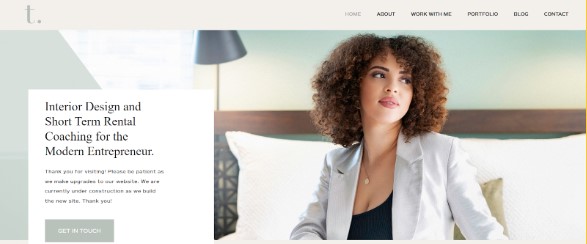The image depicts a sophisticated website homepage with a minimalist design. At the top of the page, a light gray area spans across with navigation options on the right: "Home," "About," "Work With Me," "Portfolio," "Blog," and "Contact." On the left side of this gray section, there is a lowercase "t" followed by a period. A striking gold line runs vertically down the right side of the image from top to bottom.

To the left of the gold line, a prominent white box contains the text "Interior Design and Short-Term Rental Coaching for the Modern Entrepreneur." Beneath this, there is additional text, although it's too blurry to decipher entirely, except for the word "thank you." Below this text, a gray button labeled "Get in Touch" invites user interaction.

The background reveals a cozy bedroom setting with a wooden headboard and a light blue wall. A black lamp provides ambient lighting, and decorative pillows are arranged against the headboard. The room is further personalized by the presence of a woman with curly hair, dressed in a white jacket, completing the warm and inviting atmosphere.